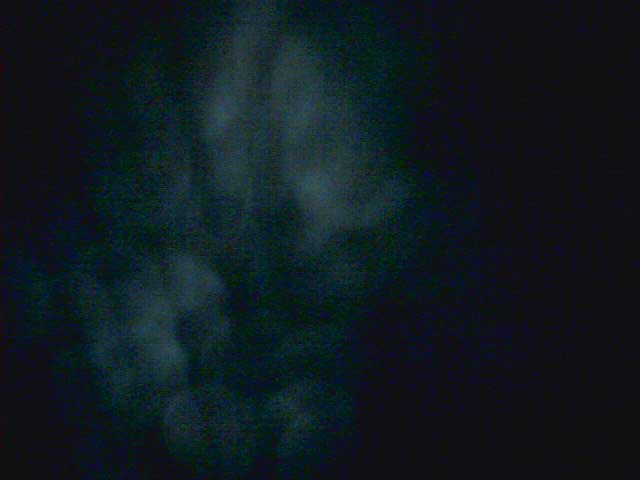The image depicts a predominantly black background with an indistinct blur of lighter patches off-center to the left, featuring hues of gray with a bluish tint, giving the appearance of ghostly, cloud-like formations. The photo is grainy and pixelated, and the light patches are characterized by eerie, almost face-like shapes that contribute to a spooky, surreal atmosphere. The lighter splotches, which are separated by areas of darkness, exhibit an ambiguous, ethereal quality, resembling smoke or a dark night sky devoid of stars. The grainy texture and color palette of blue, teal, green, and gray further enhance the mysterious and unsettling mood of the image, with some observers suggesting the faint outlines of a skull or a plant, adding to its enigmatic and creepy nature.